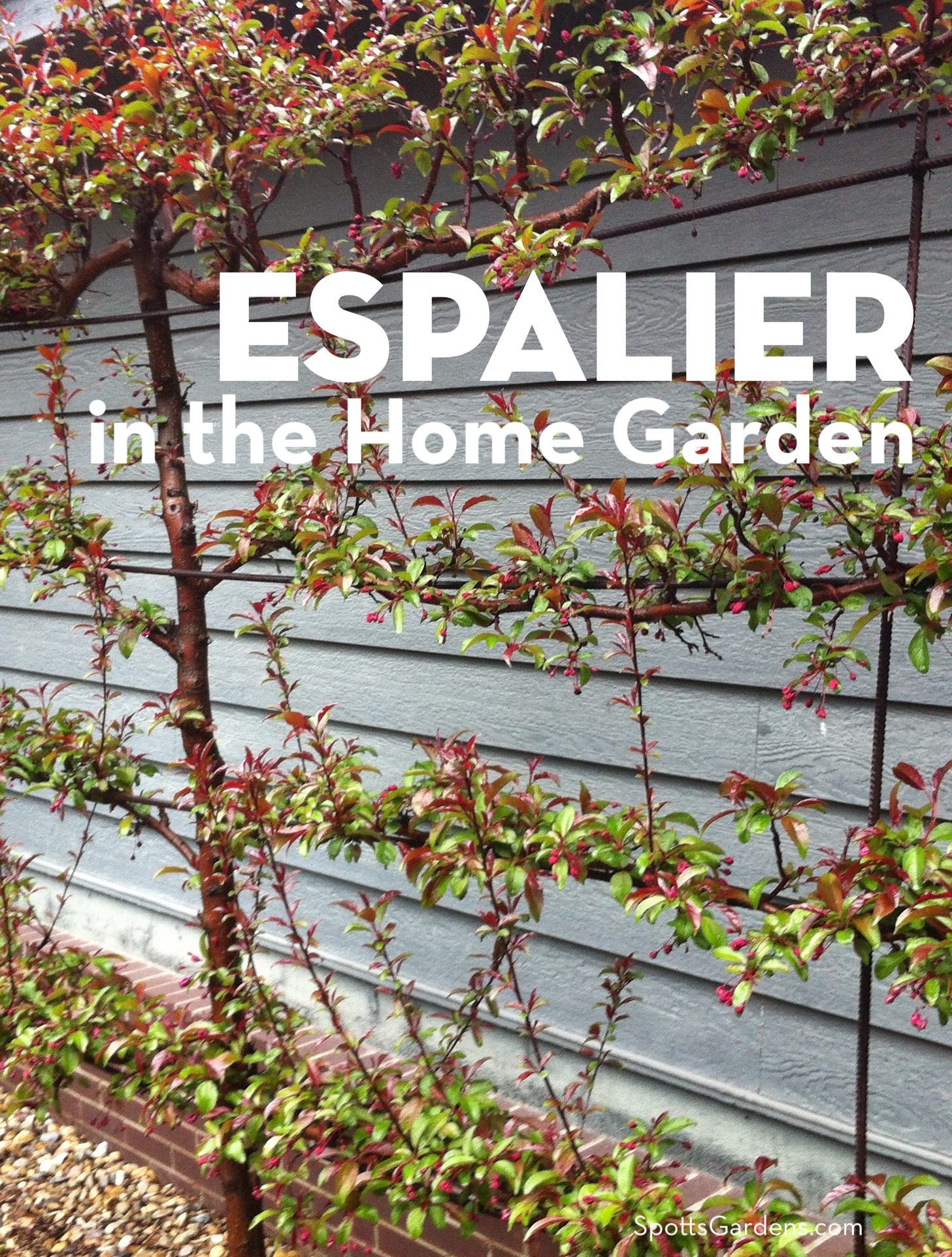This photograph, in portrait layout, showcases an espalier plant arrangement against a green fence with horizontal slats. In the foreground, there's a low brick wall reaching about calf-height, adorned by rows of various vines and plants. The plants display thin, brown stems or trunks with numerous side branches bearing green and red leaves, arranged in distinct horizontal rows along the bottom, middle, and top sections of the image. The plants seem to be supported by a wire or metal framework designed to facilitate their growth. In the middle of the picture, amidst the plants, white text reads "Espalier in the Home Garden." The backdrop of green fence and lush foliage is accentuated by the detailed arrangement of the plant's structural supports, enhancing the overall aesthetic and agricultural technique displayed.